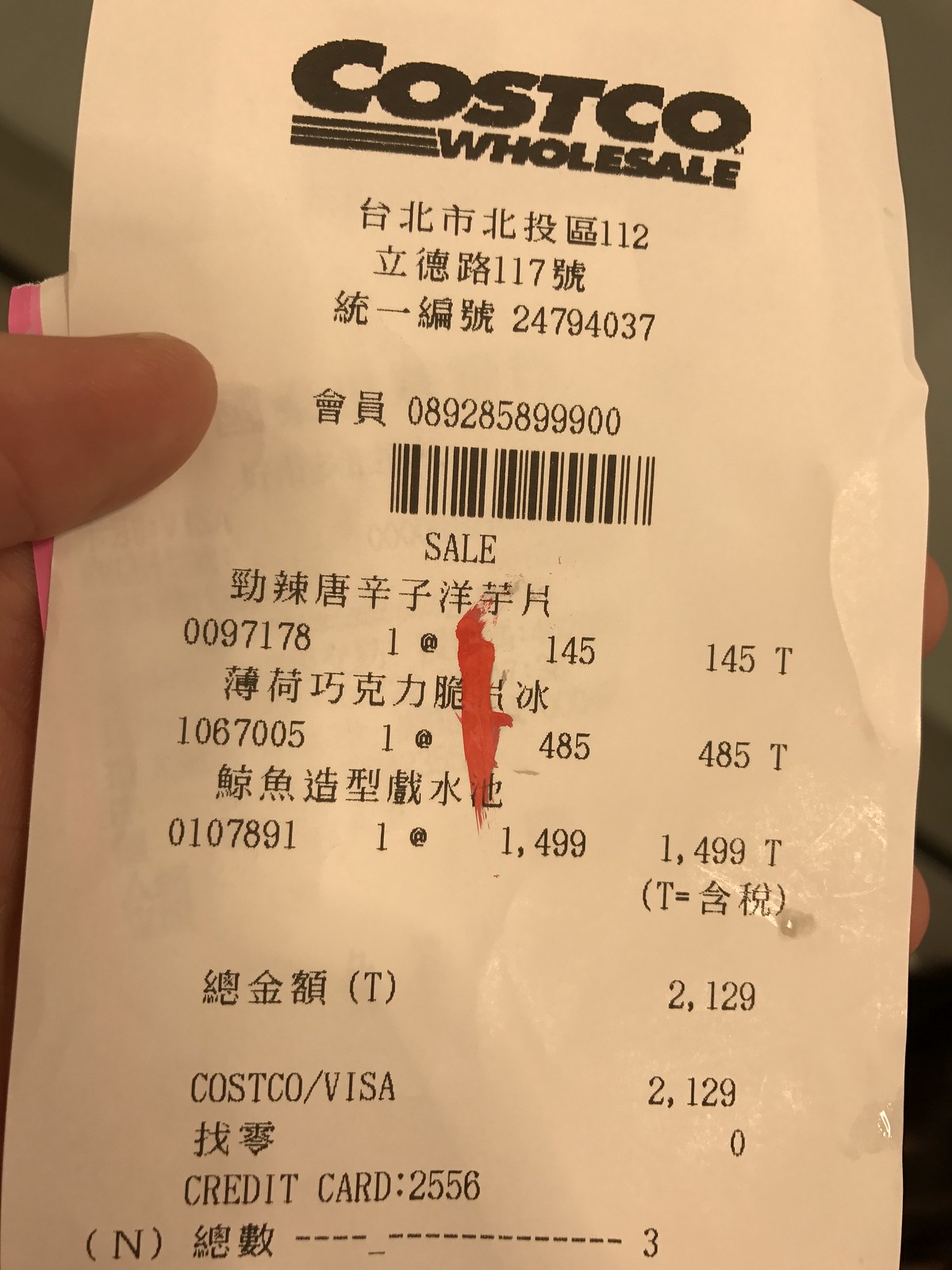A detailed caption for the image could be:

"A close-up photograph of a receipt from Costco, likely from a store in China or Japan, held by a left hand. The hand is positioned with the fingers wrapped around the receipt, just below the pointer finger. The hand is adorned with two rubber bands, one white and one pink, positioned near the palm. The receipt is typical off-white paper with black ink, featuring 'Costco Wholesale' prominently at the top, along with a mix of Arabic numerals and Chinese characters. There is a barcode and details indicating a sale, including item costs and 'Costco Visa'. The right edge of the receipt appears slightly wet. In the distant background, indistinct shades of gray and black can be seen."